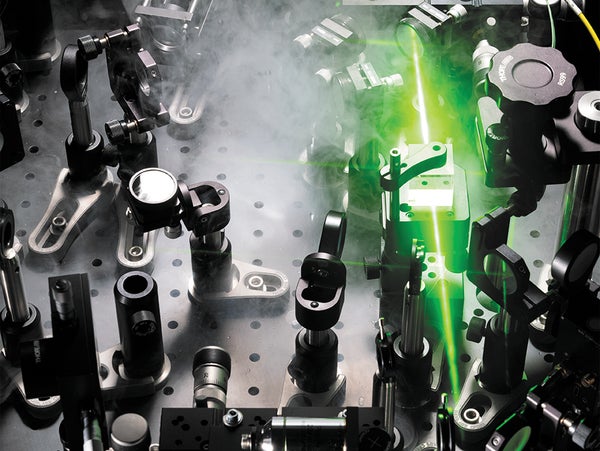The image depicts the inner workings of a complex laser mechanism set upon a gray, perforated surface. Dominating the right side of the image, a vibrant green laser projects upward, creating a smoky haze that enhances its visibility. The laser first strikes a mirror near the top, slightly right of center, and reflects to a nearby mirror on the left, following a series of precise, zigzag patterns as it ascends. The machinery is primarily composed of chrome and black components, with various instruments and vertical devices housed in systematically arranged holes on the gray base. Some components are mounted on metal bars with gray oval structures around them, suggesting mobility for adjustments. Notably, at the top right corner, there is a faintly readable white-labeled knob along with visible orange and green wires, adding to the intricate detail of the setup.